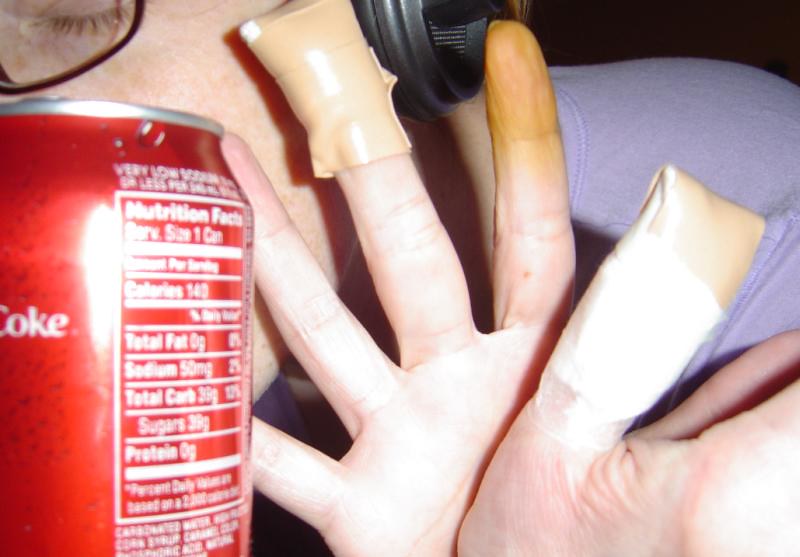A close-up photograph features the partial face and shoulder of a person wearing black headphones, dark-rimmed glasses, and a gray t-shirt. The person appears to be holding a red can of Coca-Cola prominently in the foreground, displaying the Nutrition Facts label. Visible are two hands, with one palm facing the camera and the other angled away. The thumb of the rear hand is heavily bandaged with tan tape and white gauze, while the front hand's middle finger has a tan bandage. The index finger of the same hand appears stained brown, possibly from Betadine solution. The only visible eye of the person is closed, and a bright flash creates glare on the bandages and the can, emphasizing the intricate textural details. The hands, partially obscuring the face, suggest the person might be shielding themselves from the camera or simply posing with the can.